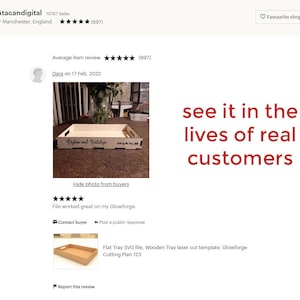Caption: 

At the top of the webpage, a gray bar spans the width with "ITACAN Digital" prominently displayed in black text on the left side. Beneath this, in gray text, it reads "Manchester, England," accompanied by five black stars and the number "807." On the top right of this gray banner, there is a button featuring a heart icon with "Favorite" inscribed next to it. 

The main content area features a clean, white background. There is text that partially reads "average something reveal five stars," followed by a user icon depicting a gray silhouette. The text beside the icon notes, "Data on 11th February 2022." 

Centered below this section is a photo, showcasing a wooden flat cart – or possibly a box with handles on each side – set on a brown ground with curtains in the background. 

On the right side of the webpage, large red text urges viewers to "See it in the lives of real customers." Directly beneath the main image, the content includes another display of five stars, and the option to "Contact buyer and post a public response now."

Below this, there is a smaller picture of the brown wooden tray, labeled "Flat Tray SVG File Wooden Tray..." with accompanying small text that isn’t legible.